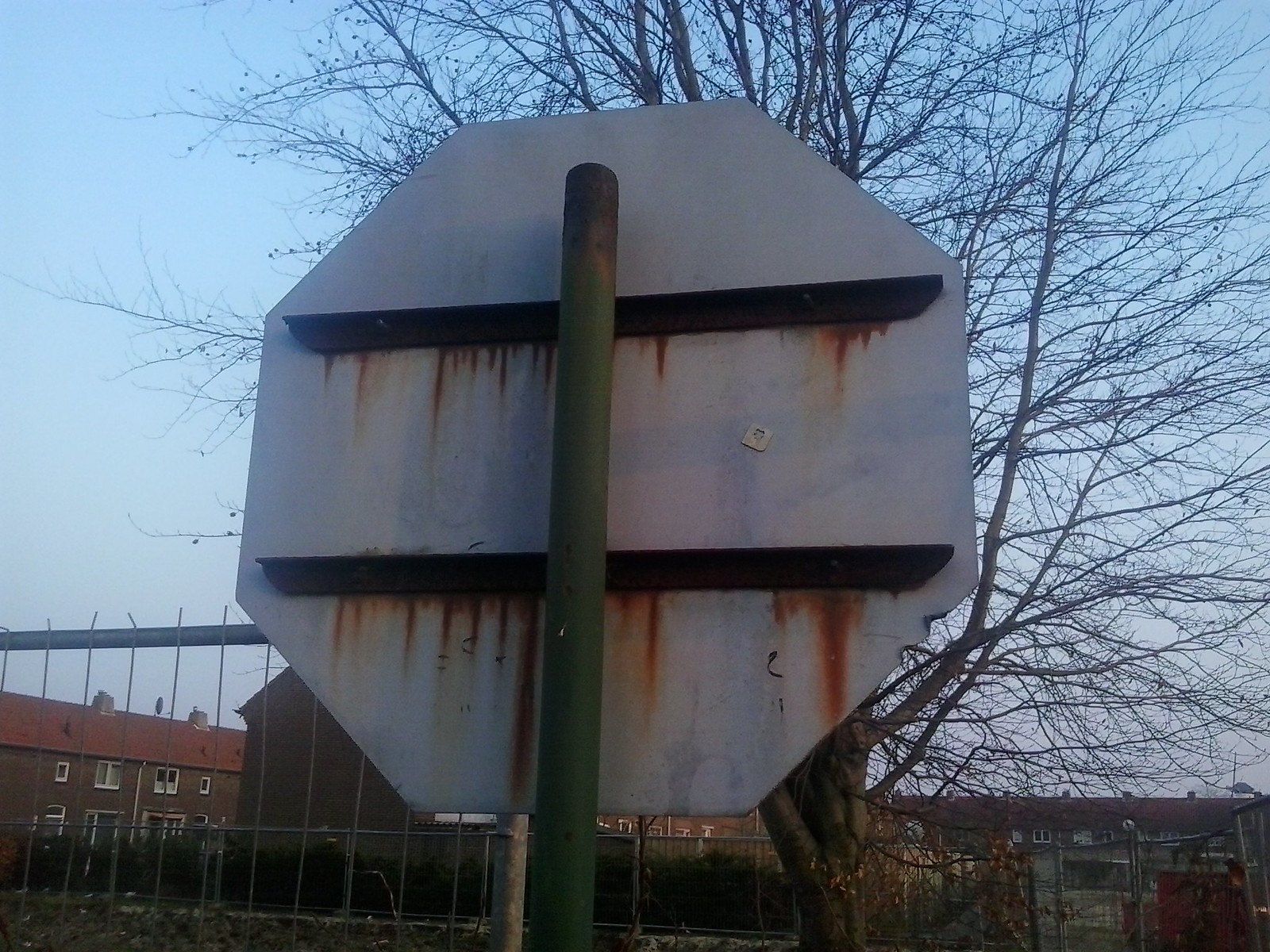This outdoor photograph captures the backside of a stop sign mounted on a dark green pole, which is attached vertically to two rusty metal support posts. The sign itself is octagonal and appears either white or silver, with distinct vertical streaks of rust running down its surface. The lighting is somewhat hazy, contributing to a slightly dim ambiance. In the background, there's a large, leafless tree, suggesting late fall or early winter, standing adjacent to a wired fence with dark-gray poles on the left. Beyond this scene, there are two prominent apartment buildings with reddish-brown exteriors and red roofs, complemented by multiple small gray chimneys peeking out. The upper half of the image is dominated by a clear, bright blue sky, visible even through the tree's bare branches, enhancing the photograph's depth and contrasting the weathered appearance of the stop sign.